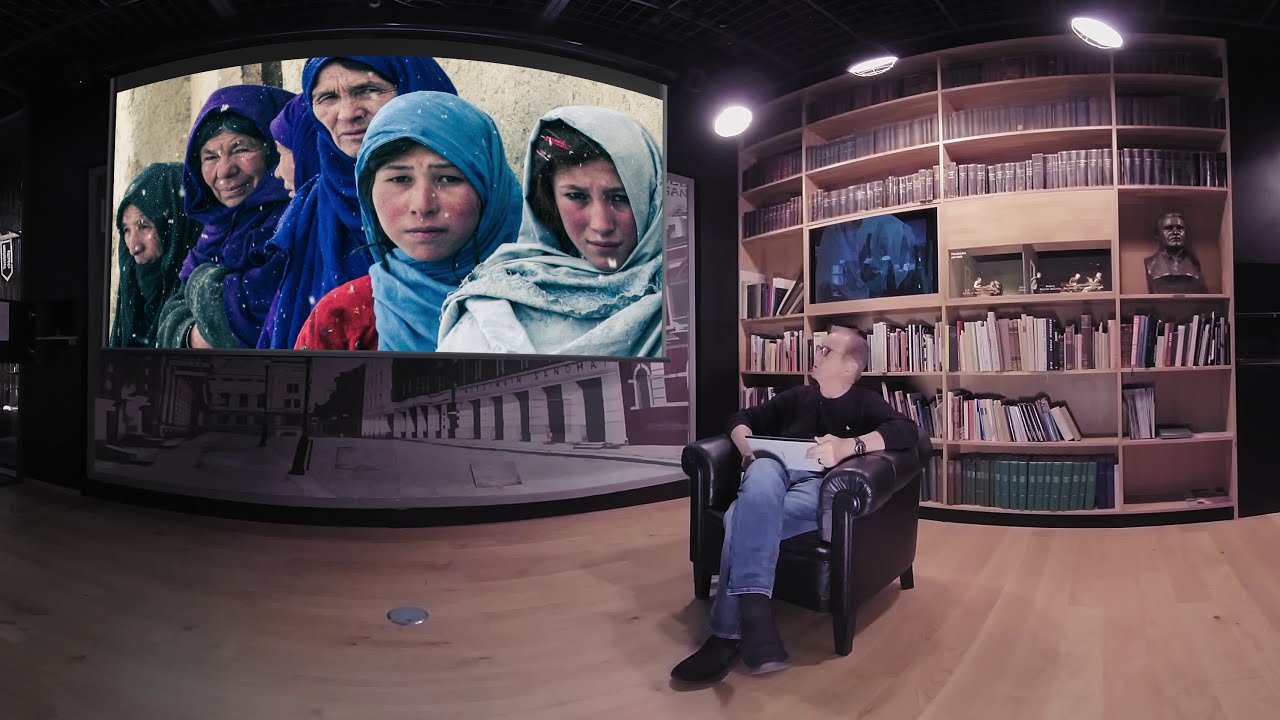In the image, a middle-aged white man with short grayish hair is seated in a leather-armchair on a wooden floor, possibly in a library or a specialized room. He is dressed in a black long-sleeve shirt, blue jeans, and black shoes, with glasses and a watch. He holds a tablet in his hand and gazes up to his left at a large, slightly curved projector screen. The screen displays an unsettling winter scene of six women and girls, all appearing distressed, with headscarves suggestive of an oppressive situation. Behind him, on the right side, is a large light-wood bookshelf filled with numerous books, a bronze bust, and some artwork. The room offers a blend of casual seating and intellectual ambiance, hinting at a scholarly or presentation setting.